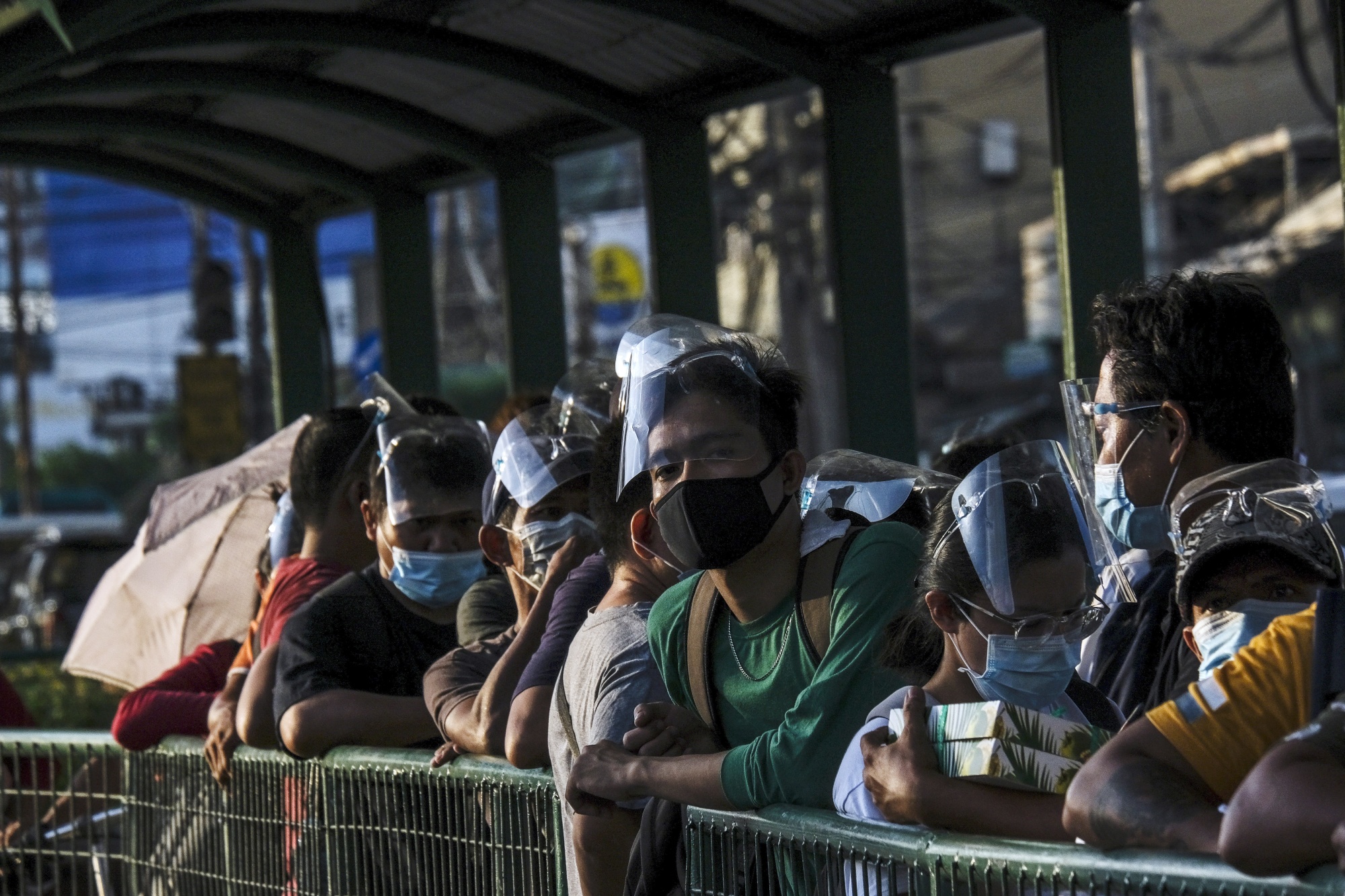The photo captures a group of people, mostly of Asian descent, gathered outdoors behind a low, green metal railing, under a canopy roof with windows. The scene is in partial shade with sunlight illuminating the group from the left side. They are all wearing masks and plastic face shields, suggesting the photo was taken during the COVID-19 pandemic. A young man with short black hair, dressed in a green long-sleeved shirt and backpack, stands in the center of the frame, directly facing the camera. Most others are leaning against the railing, gazing in different directions. The bright blue sky and distant power lines can be seen in the background.